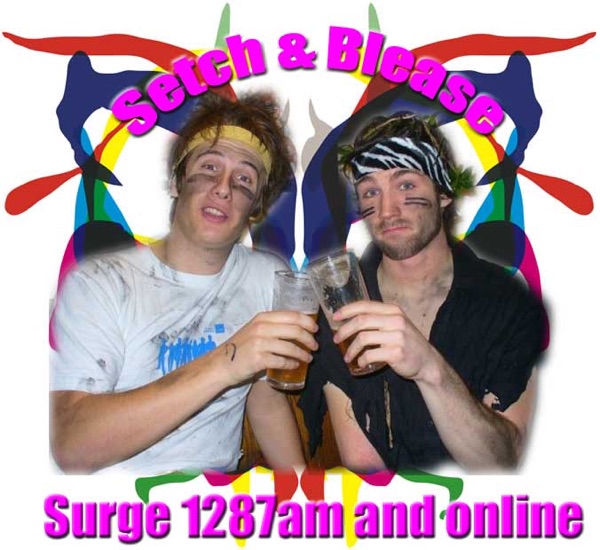In the center of the image, two men are standing shoulder to shoulder with their heads tilted slightly toward each other. They are both wearing headbands, one with a zebra pattern and the other in yellow. Both have black lines painted under their eyes, giving a rugged look enhanced by the painted or dirty appearance on their faces. The man on the left is dressed in a white shirt with a blue design, and he holds a tall glass of beer in his right hand, which is extended across his chest. The man on the right, who appears to be wearing a dark makeshift shawl, holds a tall glass of beer in his left hand. They are in the act of toasting, their glasses meeting in the center of the image. The background is predominantly white with a colorful, software-created design, featuring shades of red, green, pink, blue, yellow, black, and purple. Text overlays are present at both the top and bottom of the image, reading “Such and Bliss, Surge, 1287 AM and online.” This composition suggests the image may be an advertisement for a radio or TV show.